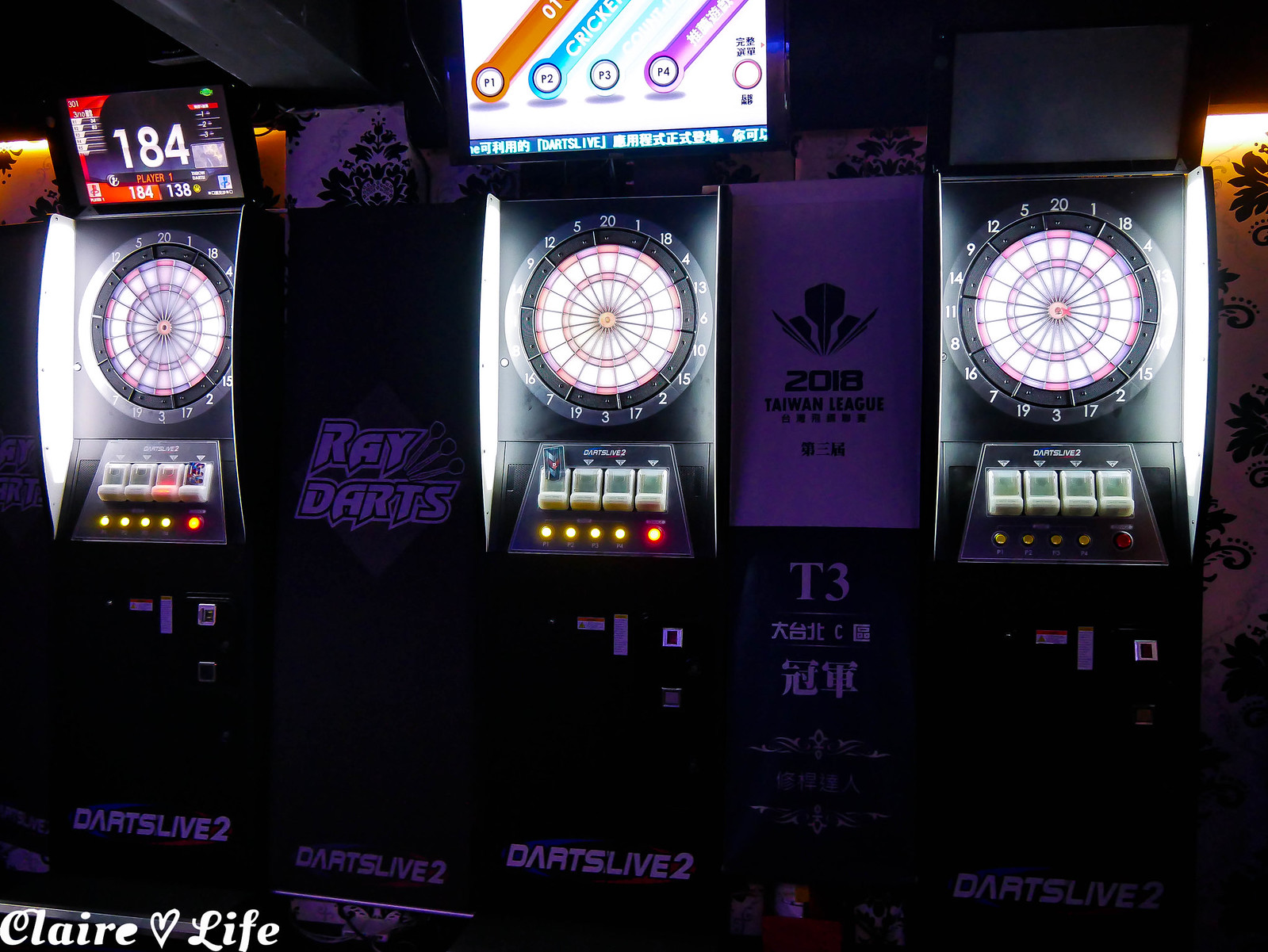This darkly lit photograph features a lineup of three electronic dart games, each framed in sleek black displays. Each display houses a standard circular dartboard in shades of red, white, and black, resembling a watch face with white numbers around its outer edge. Along the sides of each dartboard, bright white lights accentuate their prominence. Underneath each dartboard, there are four slots accompanied by a variety of glowing yellow and red buttons. Further down, at the base of each display, a metallic square-shaped coin slot is situated. The bottom of each display proudly proclaims "Darts Live 2" in white text. 

Prominent in the upper half of the image, there's a small digital screen displaying an orange, blue, and purple graphic with white background. Text on this screen reads, "P1, P2, P3, and P4," suggesting a scoreboard for players. To the left of the displays, there's black text on a white wall stating "2018 Taiwan League." Between the left and middle dartboards, another set of white text against a black background reads "Ray Darts."

In the bottom left-hand corner of the image, white text spells out "Claire Life" with a heart symbol nestled between the words. On the electronic scoreboard above the left dartboard, the number "184" is clearly visible, indicating an active game.